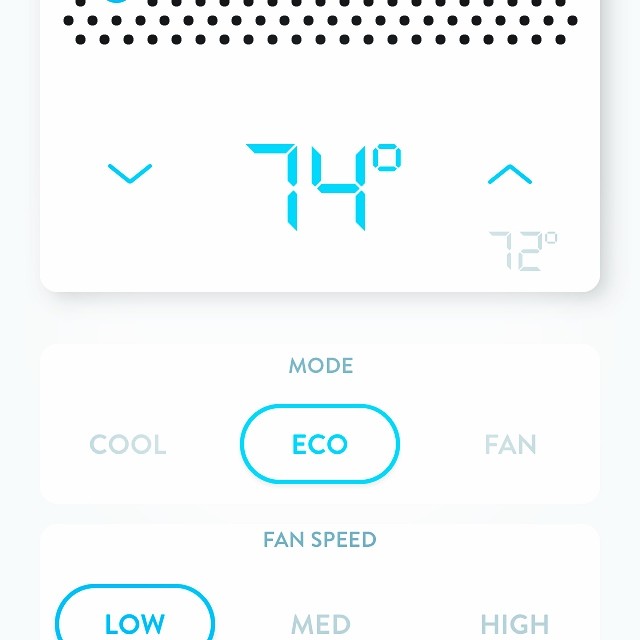The image depicts the display panel of a digital thermostat or fan control unit. At the top of the display, the temperature is set to 74 degrees Fahrenheit, presented in a blue segmented digital font. An upward-facing arrow to the right of this temperature indicates an adjustment option, while a downward-facing arrow to the left shows a lower temperature setting of 72 degrees, displayed in gray.

The upper part of the screen also features a series of black dots arranged in a pattern, likely indicating the current mode or status. Below this, the screen shows different modes with "Eco" mode highlighted. To the left of "Eco" mode is "Cool" mode, and to the right is "Fan" mode, both grayed out to indicate they are not currently active.

Further down, the fan speed setting is visible, with the "Low" option highlighted in blue, while "Medium" and "High" options are shown in gray. The section displaying the temperature is surrounded by a thin frame, distinguishing it from the rest of the controls.

The overall design is minimalistic, with a clean white background and a simple white and blue color scheme. The highlighted options stand out in blue, while inactive settings are grayed out, providing a clear and user-friendly interface.